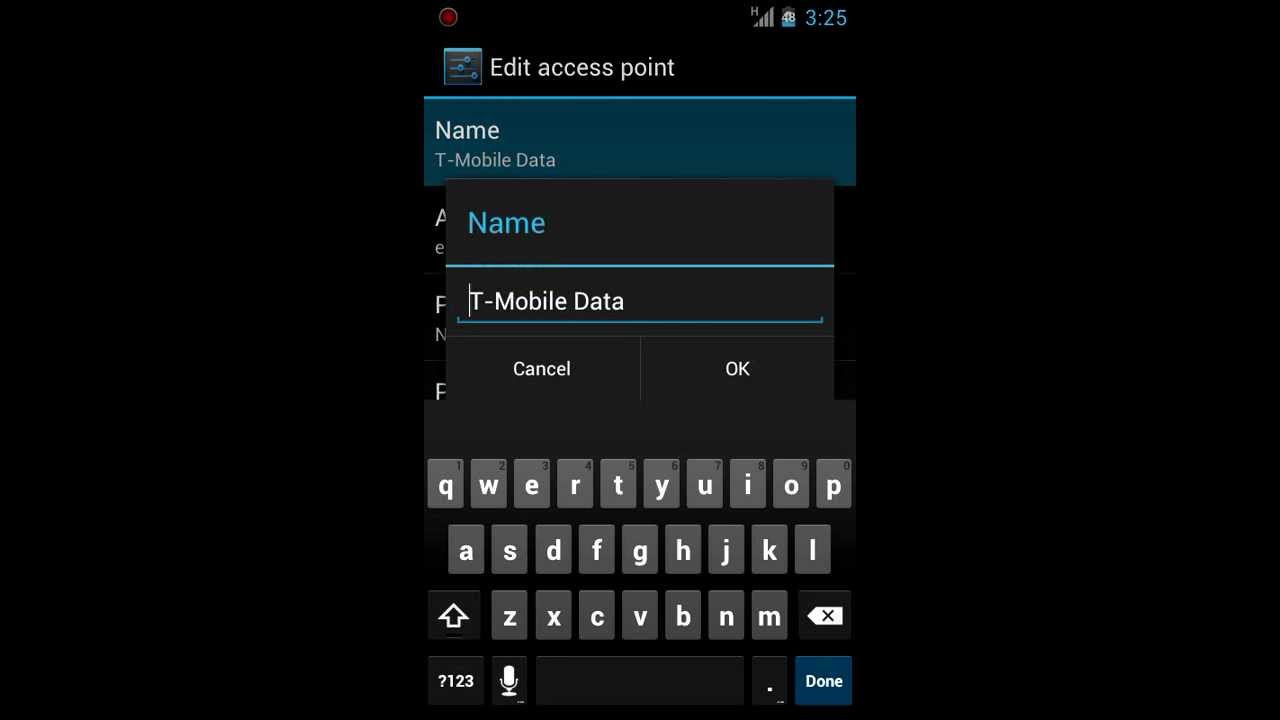The screen capture showcases an iPhone interface set in dark mode, specifically depicting the "Edit Access Points" screen. At the top of the screen, the title "Edit Access Points" is displayed. Below it, there are labeled fields starting with "Name" and followed by "T-Mobile Data." 

In the center of the screen, a pop-up dialogue is presented, reiterating the "Name" field, which again shows "T-Mobile Data" underneath. This pop-up features two buttons: "Cancel" on the left and "OK" on the right. 

The iPhone's standard keyboard is visible at the bottom, suggesting that text input for the "Name" field is active. A cursor is positioned next to the "T-Mobile Data" label within the pop-up, indicating where text would be entered.

The overall image serves as a visual guide, illustrating how users would edit an access point name for T-Mobile data on an iPhone, highlighting the user interface elements and layout in dark mode.